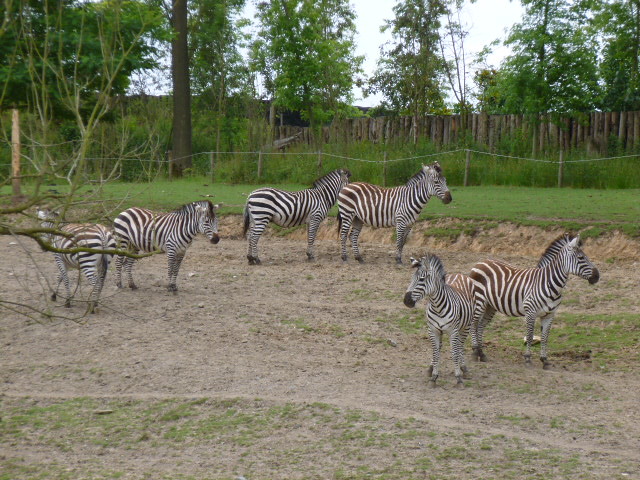The photograph captures a zoo setting showcasing the zebra exhibit under overcast skies, creating a dimly lit scene. The enclosure features multiple layers of barriers, including a foreground with line posts and wire, and a background with taller wooden fences made of columns of logs. Trees and green shrubs add depth behind these barriers, enhancing the outdoors setting. In the middle ground, six zebras, with their iconic black and white stripes, are standing on mostly bare dirt with scattered patches of grass. The zebras vary slightly in size, with two smaller ones positioned towards the bottom right and four larger ones on the top left. Overall, the environment suggests a spring or summer season, given the lush green foliage.